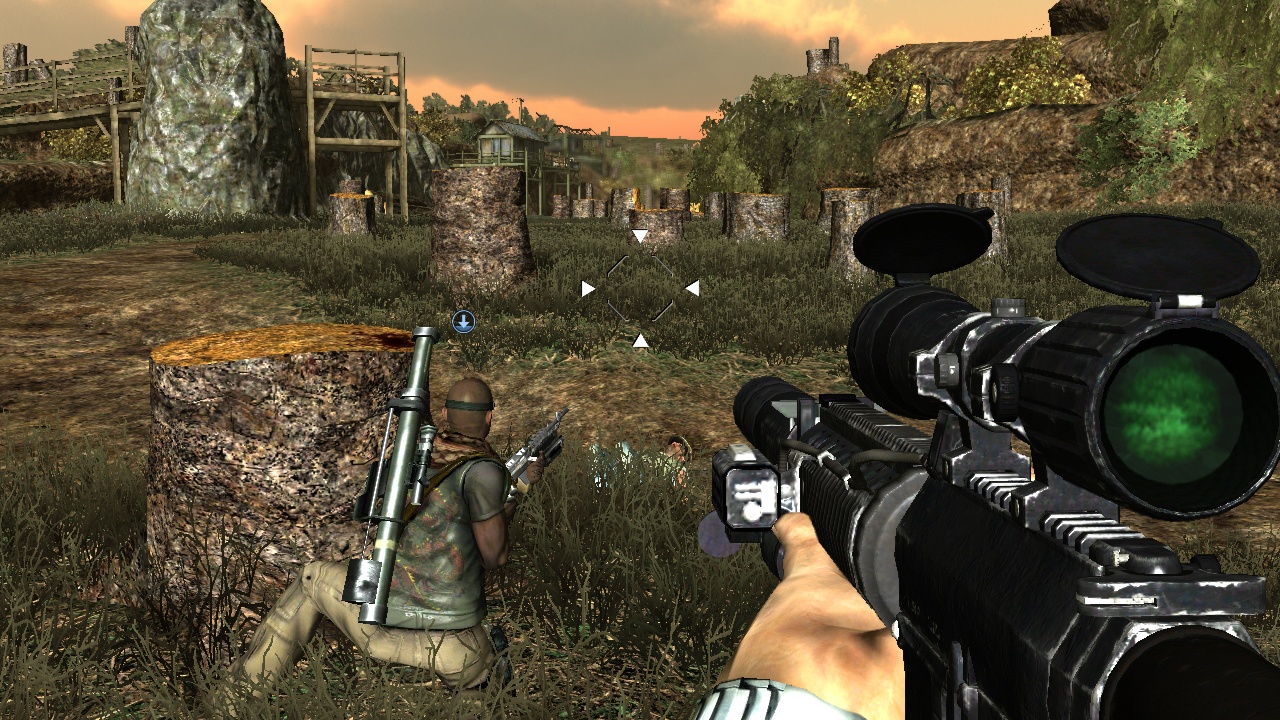In this third-person shooter game screenshot, the scene is a highly detailed outdoor setting with rocky terrain, a partly cloudy sky, and various environmental elements like wooden ladders and beams forming a bridge. In the foreground, a player's character is visible, equipped with a scoped weapon featuring a green lens. The character's arm is extended forward, and a wristwatch is visible on their hand, hinting at some level of detail in personal gear. Despite the somewhat mediocre graphics rendering of human figures, the environment is vivid with distant houses dotting the landscape. Central to the image is a targeting reticle aiming directly at an opponent who is partially concealed behind a tree stump. Additionally, there is another figure lying prone on the ground, likely a neutralized target. This tense moment captures the strategic and combative elements of the gameplay.